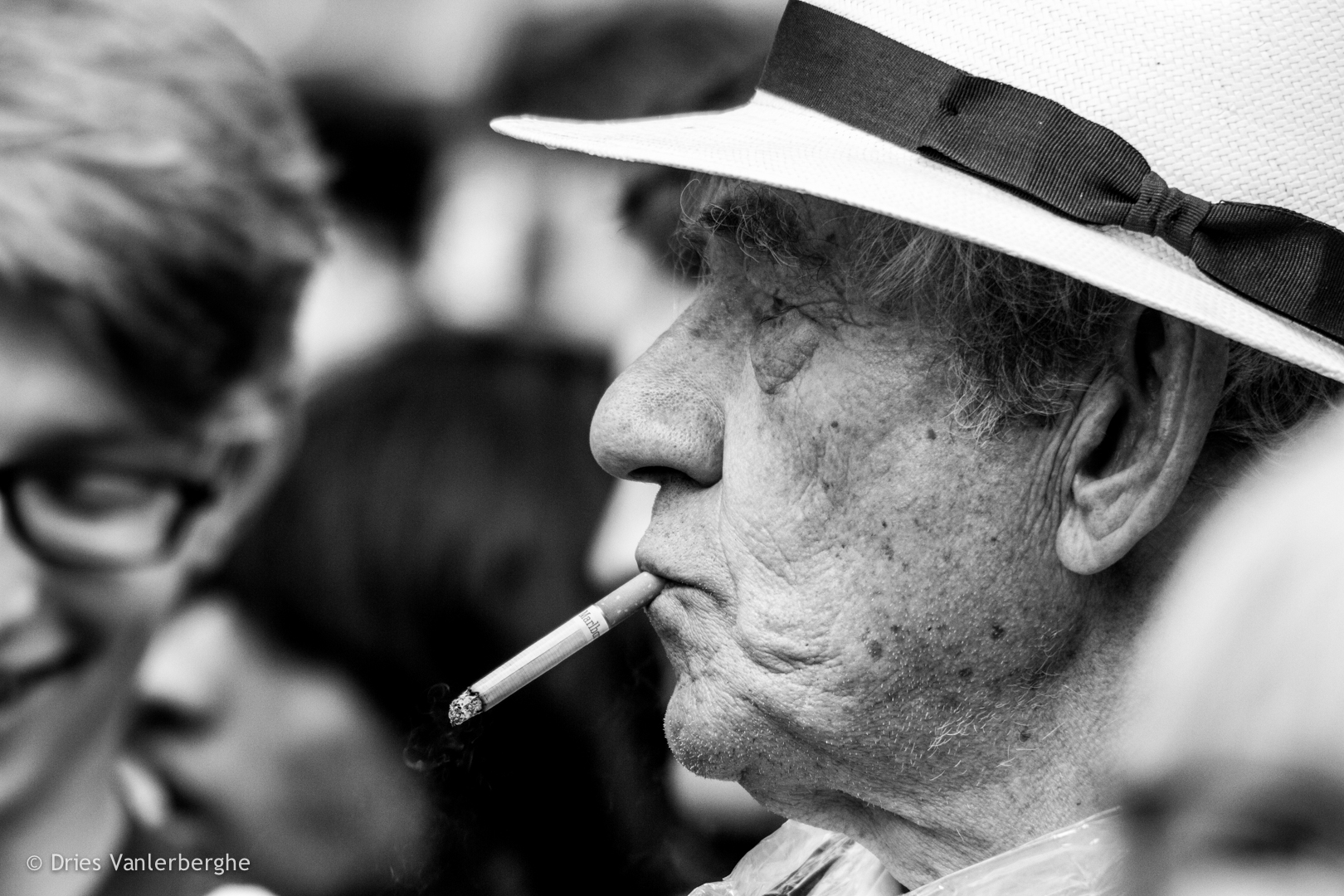This black and white photograph captures the somber profile of an elderly man, accentuating his deeply wrinkled skin, sagging features, and sun-spotted complexion. His wispy gray hair peeks out from beneath a wide-brimmed white hat adorned with a black ribbon. Dominated by bushy eyebrows, his face is depicted in exquisite detail, right down to the bags under his eyes and the cigarette burning at the corner of his mouth. The background features blurred, grayscale images of other individuals—fleeting glimpses of a nose, mouth, eye, and even a half-visible face with black-framed glasses and a toothy smile. The scene appears to be a contrast of isolation and presence, with all focus on the thoughtful and serious expression of the man. In the bottom left corner, a small text reads, "Copyright Dries Van Lerberg."